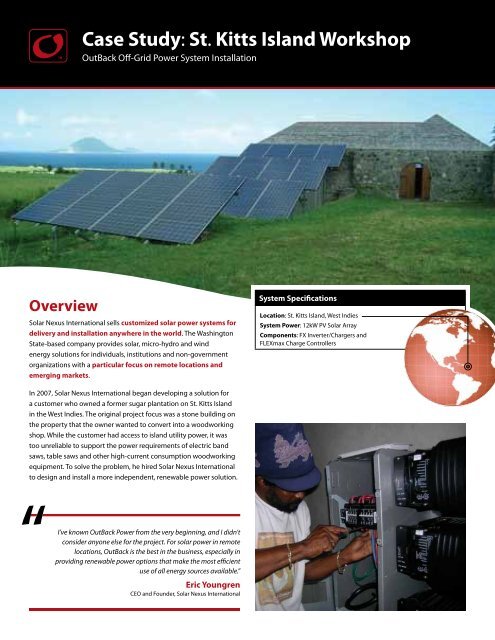This informational page serves as a case study titled "St. Kitts Island Workshop: Outback Off-Grid Power System Installation," prominently displayed in white text on a black background header. Below the header, a detailed image showcases four solar panels arranged in a semicircle formation on a lush grassy area, located in front of a stone building with a semicircular wooden door. To the man's side, there is a metal box from which large black objects are protruding. This structure is part of the former sugar plantation on St. Kitts Island in the West Indies, which a customer aimed to convert into a woodworking shop. Despite access to island utility power, its unreliability necessitated a more dependable renewable energy solution.

An overview details how Solar Nexus International, a Washington State company specializing in solar, micro hydro, and wind energy solutions for remote locations and emerging markets, was hired in 2007 to develop and install this off-grid power system. The goal was to provide sustainable energy to operate high-power consumption woodworking equipment such as bandsaws and table saws, which the unreliable island power grid could not support.

Adjacent to the image, system specifications are highlighted. These include details about the 124-watt PV solar array, FX inverters, chargers, and FlexMax charge controllers. A globe graphic indicates the installation's location on St. Kitts Island, emphasizing the global reach of Solar Nexus International's customized solar panel systems. At the bottom of the page, a smaller image depicts a man working on the installation, further illustrating the creation of this innovative off-grid power solution.